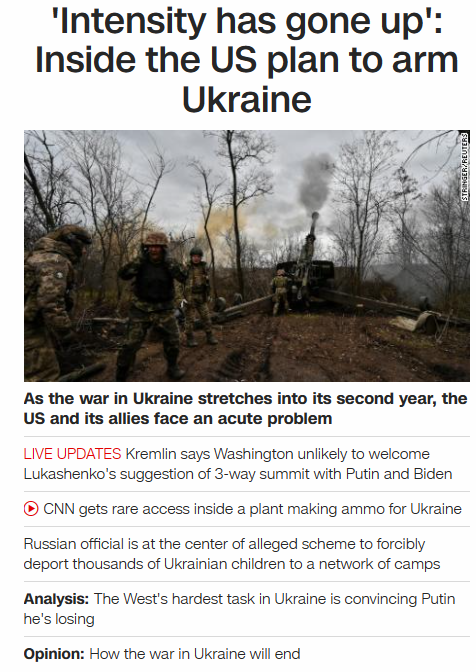**"Analysis of US Military Support for Ukraine Amidst Ongoing Conflict"**

Against a stark white background, a striking headline in large black font declares: "Intensity has increased inside the US plan to arm Ukraine." Below this headline, a photograph captures the chaos of conflict, featuring men engaged in combat, clad in army gear. The image credit "Stringer/Reuters" appears to the side among leafless trees under a cloudy sky. 

Accompanying the photograph, a text states, "As the war in Ukraine stretches into its second year, the US and its allies face an acute problem." From this point, several lines of text provide live updates and further insights:
- A red circular arrow icon introduces, "Live updates: Kremlin says Washington unlikely to welcome Lukashenko's suggestion of a three-way summit with Putin and Biden."
- The next line, marked "CNN," notes: "CNN gets rare access inside a plant making ammo for Ukraine."
- Another update reveals, "Russian officials at the center of alleged scheme to forcibly deport thousands of Ukrainian children to a network of camps."
- This is followed by a bold "Analysis" tag introducing: "The West's hardest task in Ukraine is convincing Putin he's losing."

Finally, a bolded "Opinion" segment suggests: "How the war in Ukraine will end."